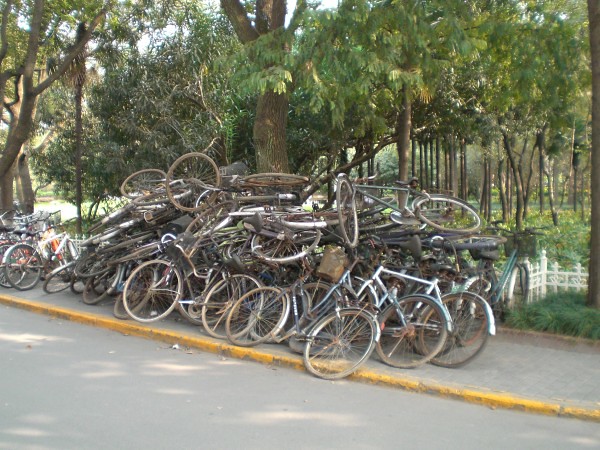This color photograph, taken on a bright day, captures an outdoor scene in what appears to be a park. The foreground features a street bordered by a painted yellow curb and a sidewalk, on which rests an enormous, disordered pile of approximately 50 adult-sized, brown, old, and tarnished bicycles. The base layer of bicycles lies on their wheels, forming a kind of foundation, with additional bicycles haphazardly piled on top, some bent and seemingly unusable. To the left, a bicycle rack contains several bicycles in good condition, neatly lined up. The background reveals a tranquil setting of grass and numerous trees, along with the presence of a pond or lake, enhancing the picturesque park setting. The overall impression is one of bicycles either discarded or left in disarray, possibly suggesting abandonment or the aftermath of some event.